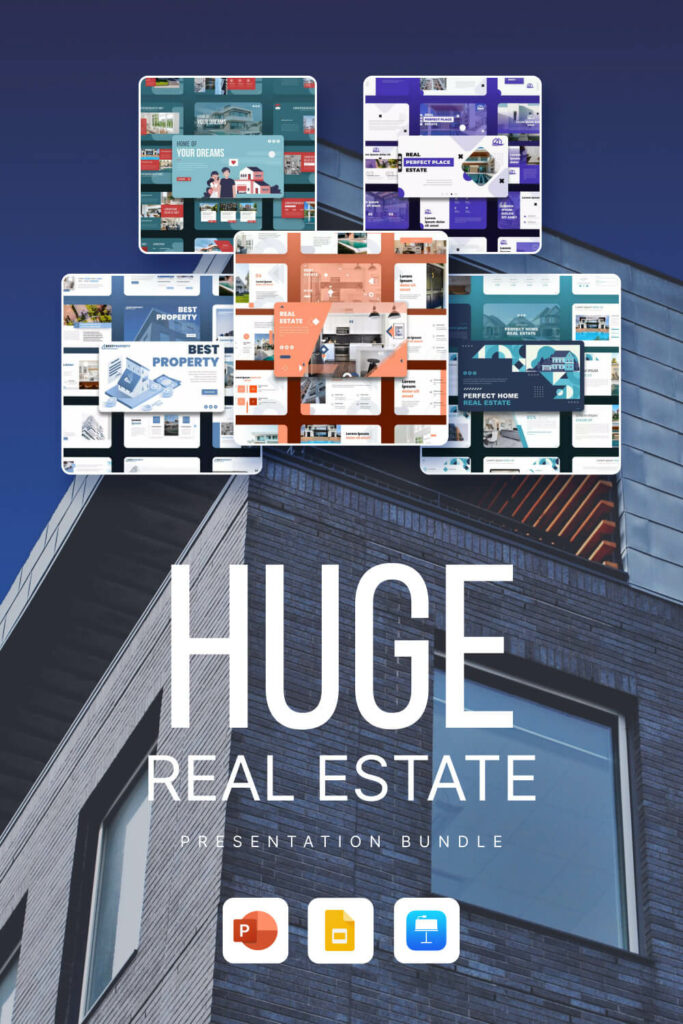The digitally generated image features a comprehensive real estate presentation bundle set against the backdrop of a modern house, captured from a corner angle. Dominating the center of the image is bold text reading "HUGE REAL ESTATE PRESENTATION BUNDLE," with "HUGE" prominently displayed in much larger font. At the bottom, icons indicate that the bundle includes a PowerPoint presentation, an interactive file, and an Excel spreadsheet. Additionally, five smaller, digitally generated images are positioned at the top, showcasing various other presentation bundles with titles such as "BEST PROPERTY," "REAL PERFECT PLACE ESTATE," "PERFECT HOME REAL ESTATE," and "THE HOME OF YOUR DREAMS," highlighting the different features and contents each bundle offers.